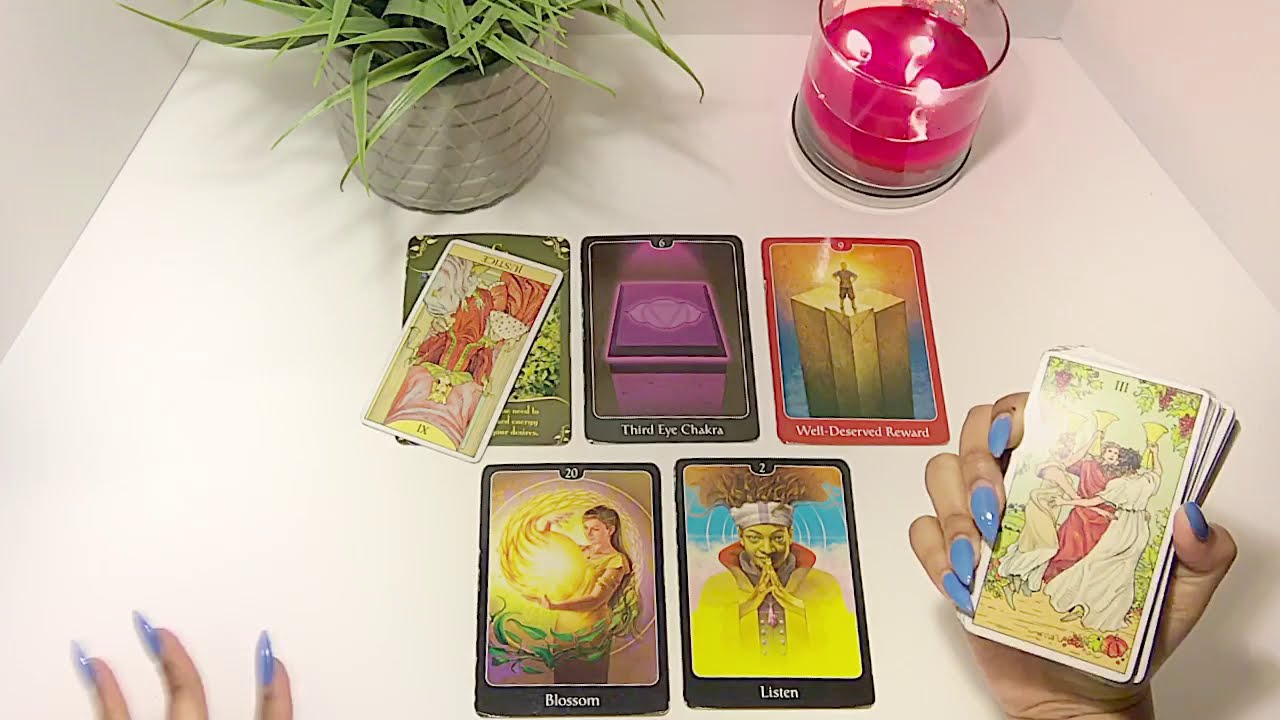This image features a white table or shelf against white walls visible in the upper corners. At the top of the table, a potted plant in a silver pot with gold stripes adds a splash of green with its long leaves. To the right sits a dark pink candle, half-filled, and glowing with three flames. Centered on the table are five cards arranged in two rows. In the top row, one card is tilted sideways on the left, while clear text on the cards reads "Third Eye Chakra," "Well Deserved Reward," "Blossom," and "Listen." The cards, adorned with colorful illustrations and words, evoke a tarot or psychic reading scenario. In the lower part of the image, a woman with long blue nails—visible on both her hands—appears to be engaged with the cards, holding a deck in her right hand and her left hand's fingers slightly blurred.